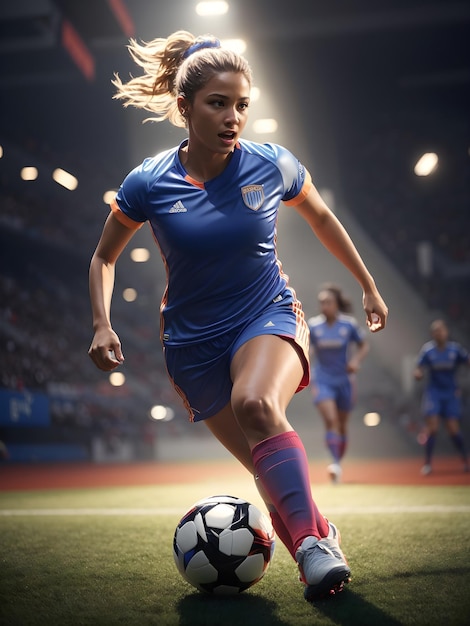A professionally taken photograph captures the dynamic energy of a soccer match, centering on a female player in mid-action. The athlete is captured in a forward sprint, leaning towards her right side with intense focus. She wears a vivid blue t-shirt adorned with symbols on the chest and matching blue shorts accented with bold red stripes along the sides. Her socks are a striking blend of red and pink, complementing the pristine white soccer cleats she sports. Positioned at her feet, a visually striking black, white, and blue soccer ball suggests her next move. 

The background, masterfully blurred to highlight the primary subject, hints at the bustling ambiance of the scene. Behind her, at least two additional soccer players are discernible, engaged in play, while a densely packed grandstand filled with spectators reflects the light, indicating a high-energy, crowded event. The playing surface is dual-toned; the immediate green grass she strides on contrasts with the reddish dirt further back in the field, where the other players are stationed. This captivating image perfectly encapsulates the competitive spirit and vibrant atmosphere of a live soccer match.